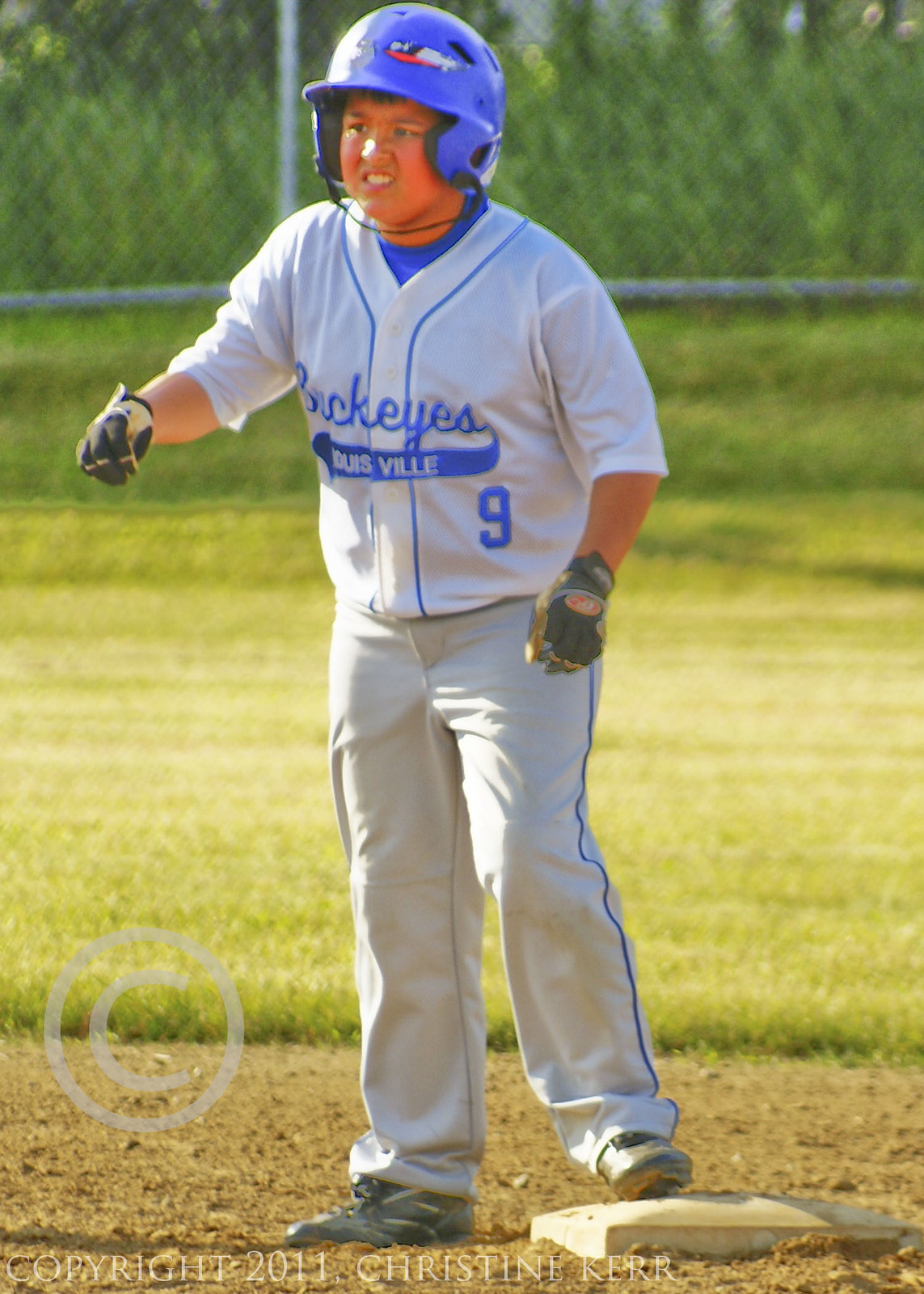The photograph captures a young baseball player poised on a base in an outdoor field. The field features a dirt infield leading to a grassy outfield and a chain-link fence, behind which are several green trees. The boy stands with one foot on the base, suggesting he is contemplating a steal. He wears white baseball pants with a royal blue stripe, a white jersey with royal blue lettering spelling 'Buckeyes Louisville' and the number 9, and a royal blue t-shirt underneath. His uniform is complemented by black batting gloves and black sneakers, and he dons a royal blue batting helmet. The boy appears to be gritting his teeth in focus. Overlaid on the bottom left of the image is a prominent copyright symbol and the text 'copyright 2011, Christine Kerr' in faint white lettering.